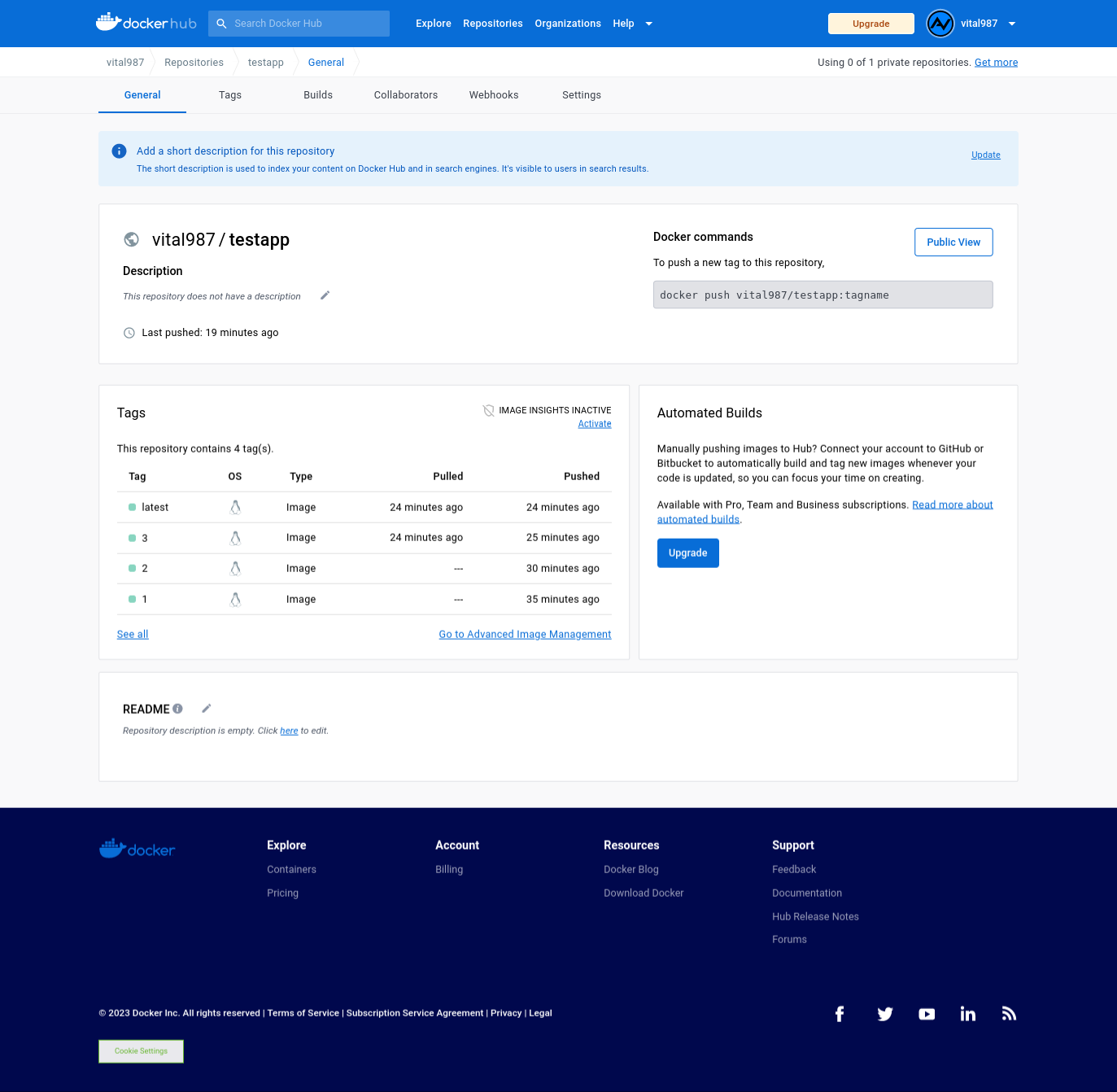**Detailed Descriptive Caption for Docker Hub Webpage Screenshot:**

The screenshot showcases a Docker Hub webpage, a popular platform for sharing containerized applications. The Docker Hub interface features a blue top bar adorned with the Docker logo, which creatively depicts a whale carrying cargo containers.

At the top of the page, navigation buttons include options such as Explore, Repositories, Organizations, Help, and Upgrade. A user avatar and a drop-down menu are positioned on the right side of the bar. The current user "Vital 987" is prominently displayed.

Below the navigation bar, the main panel highlights various repository sections for "Vital 987". Key sections include Repositories, Test Staff, General, Tags, Builds, Collaborators, Webhooks, and Settings. Each section is easily accessible via labeled buttons.

The main repository titled "Vital 987/Test App" lacks a description, essential for indexing and visibility in search results. An entry indicates the last push to this repository was made 19 minutes ago. Detailed Docker commands for pushing a new tag to the repository (e.g., `docker push vital987/testapp:tagname`) are provided.

In the central area, repository tags such as "latest," "321", "OS," etc., are listed with timestamps indicating recent pull and push activities (e.g., pulled 24 minutes ago, pushed 24, 25, 30, and 35 minutes ago).

On the right panel, links guide users to advanced image management, manual and automatic build instructions, and repository settings. A call-to-action button invites users to upgrade and access more extensive features.

Finally, the footer, set against a dark blue background, reiterates Docker branding with links to Explore, Account, Resources, and Support. Social media icons for Facebook, Twitter X, and YouTube are conveniently placed on the right. The Docker Hub page is a detailed, technical interface aimed at proficient users managing containerized applications.

**Note:** Screenshot is complex and designed for advanced technical users to manage their Docker repositories effectively.